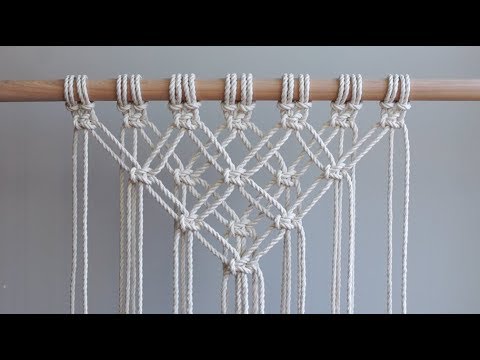This detailed screen capture depicts an intricate macramé project in progress. The image features a long, round, wooden rod positioned horizontally at the top, secured within a wide black border, and set against a grey background. Suspended from the rod are multiple sections of braided rope arranged to form an upside-down triangular pattern. The design includes a prominent X shape in the middle, accented by a flower knot. The craftsmanship highlights artistic knots and twists, resulting in seven distinct sections that contribute to the complex structure. Additional strands of rope dangle freely below the completed portion, suggesting ongoing work on this elaborate decoration that resembles a triangular wind catcher. Shadows cast by the knots and ropes add depth to the composition, emphasizing the meticulous detail and texture of the handwoven creation.